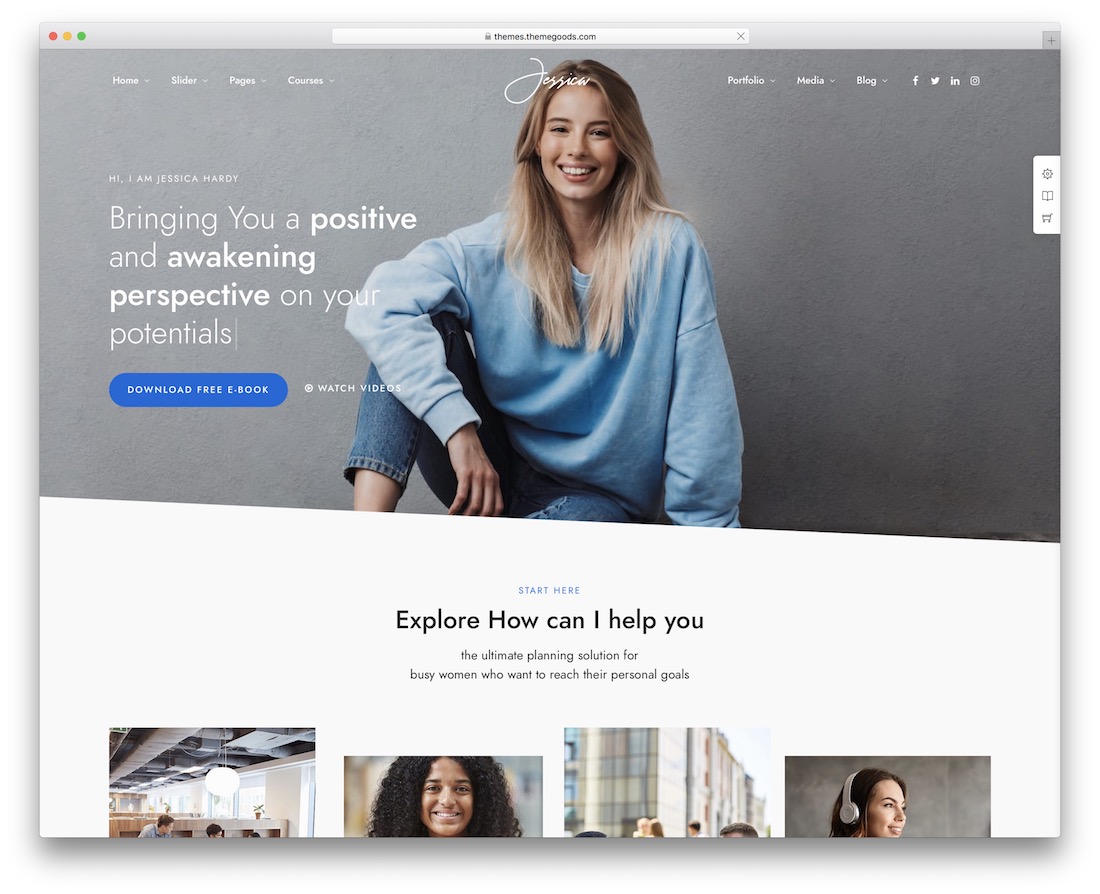The displayed webpage, found at themes.themegoods.com, features a header image of a person with long blonde hair, clad in jeans and a large blue sweater. The name "Jessica" is stylishly written in cursive white text atop this header. The navigation menu includes tabs labeled Home, Slider, Pages, Courses, Portfolio, Media, and Blog. Additionally, the page displays social media icons for Facebook, Twitter, Indeed, and Instagram.

Central to the page is an introduction that reads: "Hi, I am Jessica Hardy, bringing you a positive and awakening perspective on your potential." There is a conspicuous blue button inviting users to download a free ebook, alongside an option to watch videos.

A "Start Here" section encourages users to explore how Jessica can assist them, stating: "The ultimate planning solution for busy women who want to reach their personal goals." Surrounding this informative text, various images are featured: one depicts a workspace, another shows a woman standing at what appears to be her job, and a third captures a person wearing headphones and smiling, conveying a friendly and engaging atmosphere.